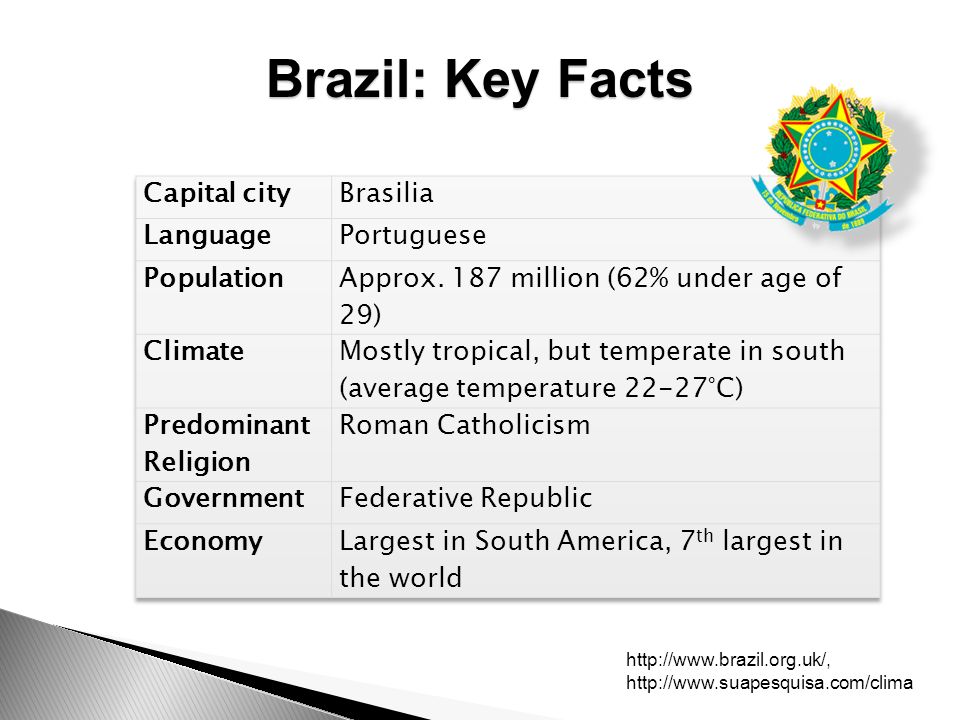This is a detailed screenshot containing key facts about Brazil from an unknown source. At the top, the heading reads "Brazil Key Facts." 

On the right side of the image, there is a graphic of a green and yellow five-pointed star. In the center of the star, a blue circle is adorned with white stars. Behind the star, a laurel wreath adds to the decorative design. Beneath this emblem, a banner displays the inscription "República Federativa do Brasil."

The central section of the screenshot provides extensive information:
- **Capital City:** Brasília 
- **Language:** Portuguese 
- **Population:** Approximately 187 million, with 62% under the age of 29 
- **Climate:** Mostly tropical, but temperate in the south with an average temperature ranging from 22 to 27 degrees Celsius 
- **Predominant Religion:** Roman Catholicism 
- **Government:** Federative Republic 
- **Economy:** The largest in South America and the seventh largest in the world

At the bottom of the image, web addresses for further information are listed: http://www.brazil.org.uk and http://www.suapesquisa.com. Also visible is the word "CLIMA," indicating the climate information section.